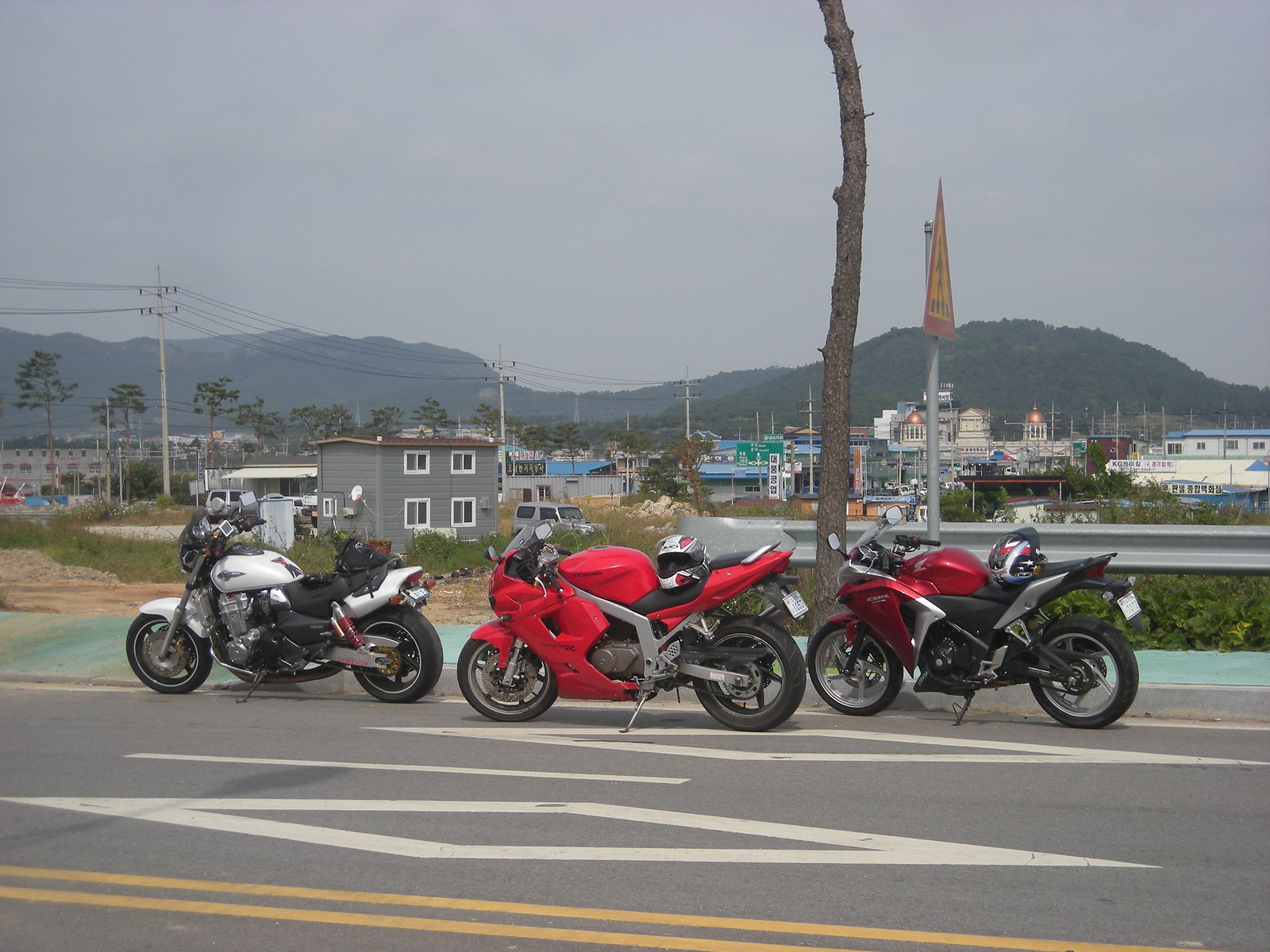This photograph captures a group of three motorcycles parked slightly in the far lane of a two-lane highway marked with HOV lane diamonds. The motorcycles are upright with their kickstands down, each sporting a helmet on their seats: a silver-red-black helmet with a dark visor on the darker red and black motorcycle at the back, a white-silver-red helmet with a clear visor on the scarlet red bike in the middle, and a motorcycle in front with a black leather seat resembling a classic police cruiser. In the background, a tree without foliage stands along the roadside next to some metal railings. Further beyond, the scene transitions into a grassy area with scattered buildings, among them a domed structure akin to a state capitol, set against a backdrop of low mountains. There are also signs of a seaside town, with boats and beachy structures near the coastline, framed by misty hills under a light gray sky.